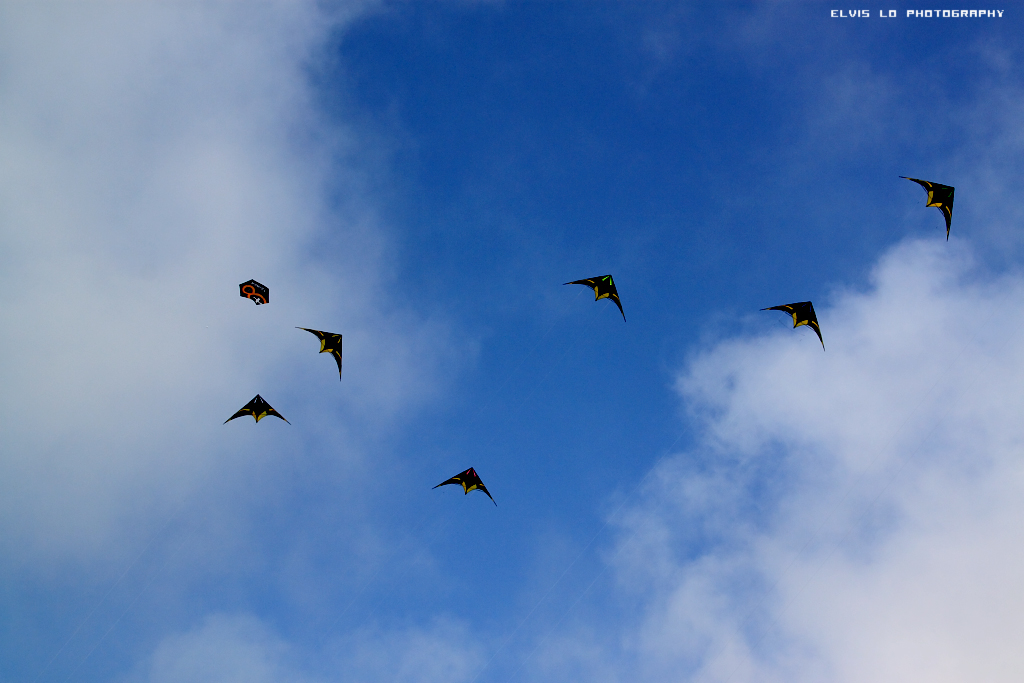This is a rectangular photograph capturing a stunning blue sky adorned with fluffy white clouds. The clouds frame the image from the sides and bottom, leaving a clear blue center. The upper right corner bears white text, too small to read but identified in one description as saying "Elvis L.A. Photography." In this serene sky, there are seven black kites, each designed with a green stripe at the front and yellow stripes towards the back, resembling the shape of a manta ray with pointy wings facing upward and to the right. Among the kites is an ambiguous object on the left, possibly another bird or a different-shaped kite.